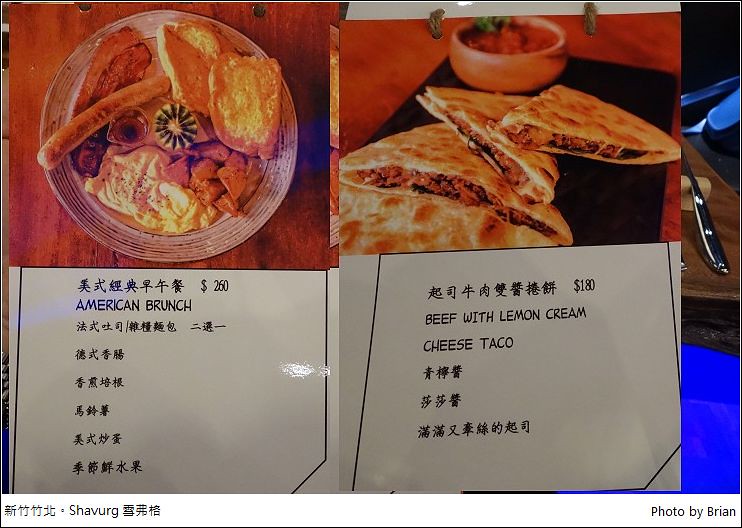This image features a two-part photo of a menu and its corresponding dishes. The menu is partially in English, printed in capital letters, and includes oriental characters, which appear to be either Japanese or Korean as we move down the menu. A price listed is $2.60, but the exact currency is unclear due to the foreign symbols preceding it. Below the price and the initial listing in the foreign script, it reads "American Brunch."

The left image showcases a beautifully rustic, handmade plate with intricate edging and striping. On this plate are two slices of bread, a sausage, a strip of bacon, and a small container of dipping sauce. Additionally, the plate includes stir-fried chunky potatoes and scrambled eggs garnished with coarse ground black pepper.

The right image highlights "Beef with Lemon Cream Cheese Taco," priced at $1.80, although the currency may differ. This dish consists of taco-style flat shells filled with beef, lemon cream, and cheese. In the backdrop, a bowl containing a garnished condiment is visible, and to the right, you can spot a table adorned with a utensil. The setting includes a blue hue in the foreground.

In the lower left corner, the word "SHAVURG" is printed, and the photo credit "Photo by Brian" is noted in the lower right corner.